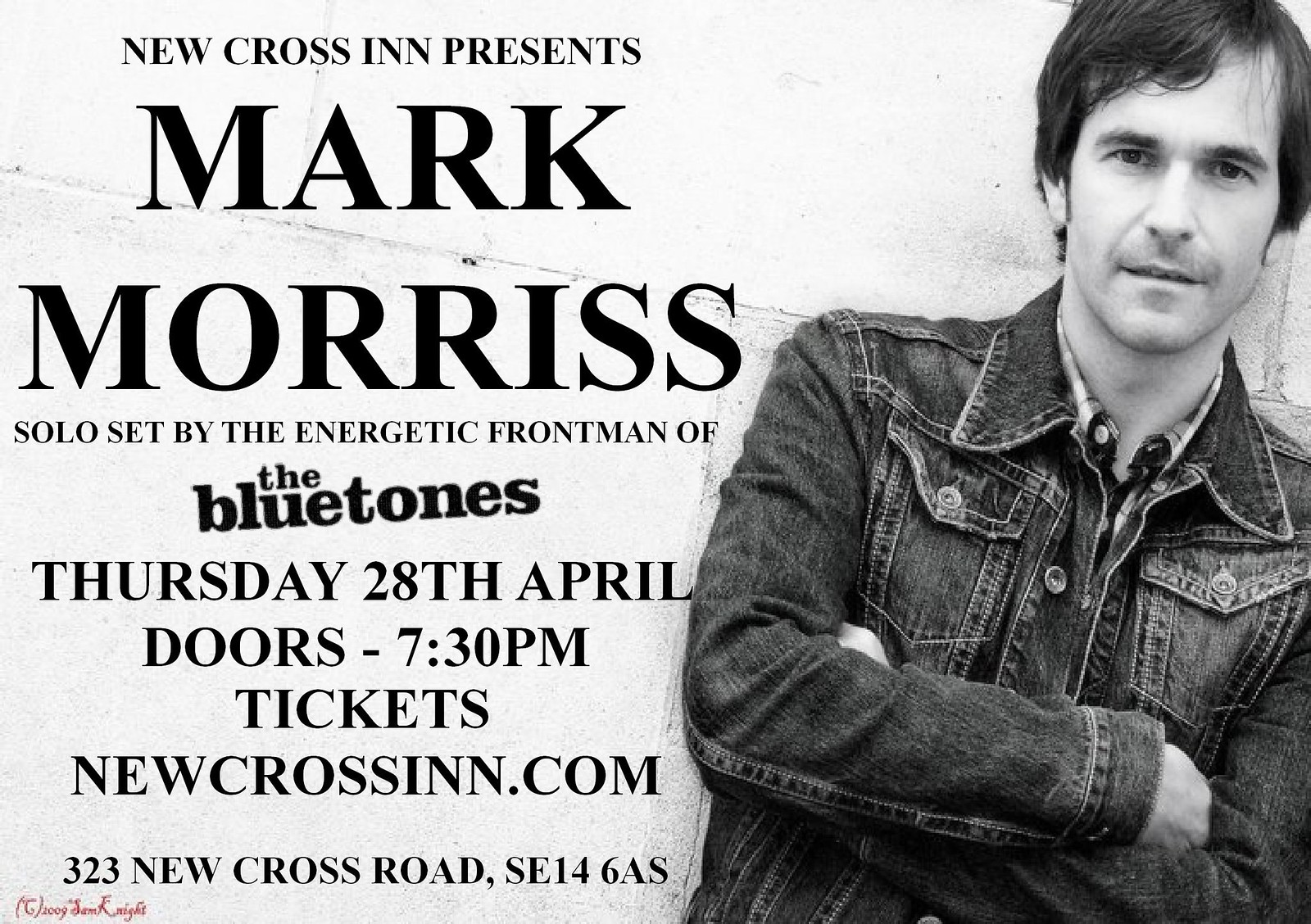The image depicts a promotional poster featuring a young white man positioned on the right side, dressed in a denim jacket over a collared shirt, with his arms folded across his chest. He has a full head of brown hair and is captured in black and white, facing the viewer. The left side of the poster contains bold black text on a white and gray background that reads, "New Cross Inn presents," followed by "Mark Morris" in larger letters. Below, it states, "solo set by the energetic frontman of The Bluetones." Further down, the text indicates, "Thursday, 28th April, Doors 7.30 p.m., Tickets: newcrossinn.com, 323 New Cross Road, SE14 6AS." Additionally, there is blurred cursive red lettering in the bottom left corner.